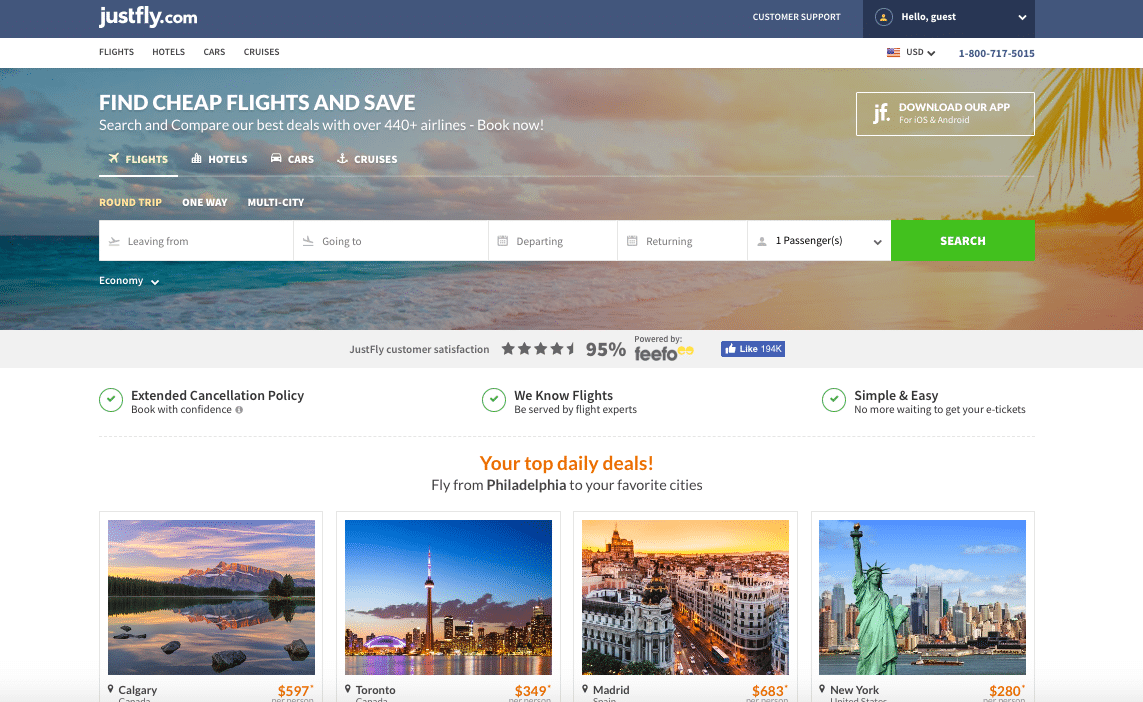The image depicts a webpage from justfly.com, a platform for booking flights, hotels, cars, and cruises. At the top of the page, there is a blue banner that includes the justfly.com logo and a customer support drop-down box. Adjacent to this, there's an icon of a person next to the greeting “Hello, Guest.” Below the banner, there's a prominent message inviting users to "Find cheap flights and save," along with a prompt to "Search and compare our best deals with over 440+ airlines" followed by a "Book Now" button.

The main navigation bar features tabs for "Flights," "Hotels," "Cars," and "Cruises," with the "Flights" tab highlighted in yellow, indicating it is currently selected. Options for trip type include "Roundtrip," "One-way," and "Multi-city," with "Roundtrip" currently chosen. Beneath these options is a search bar where users can input their departure city, destination city, departure date, return date, and the number of passengers. There is a green "Search" button to execute the search query.

Towards the bottom of the page, there are four featured travel deals, each accompanied by an image and a price. The first deal is for Calgary at $597, illustrated by a picture of a mountain. The second deal features Toronto, Canada, showcasing a city skyline. The third deal is for Madrid, with a cityscape image. The fourth deal is for New York City, highlighting an image of the city and the Statue of Liberty. These deals provide visual and pricing information to entice prospective travelers.